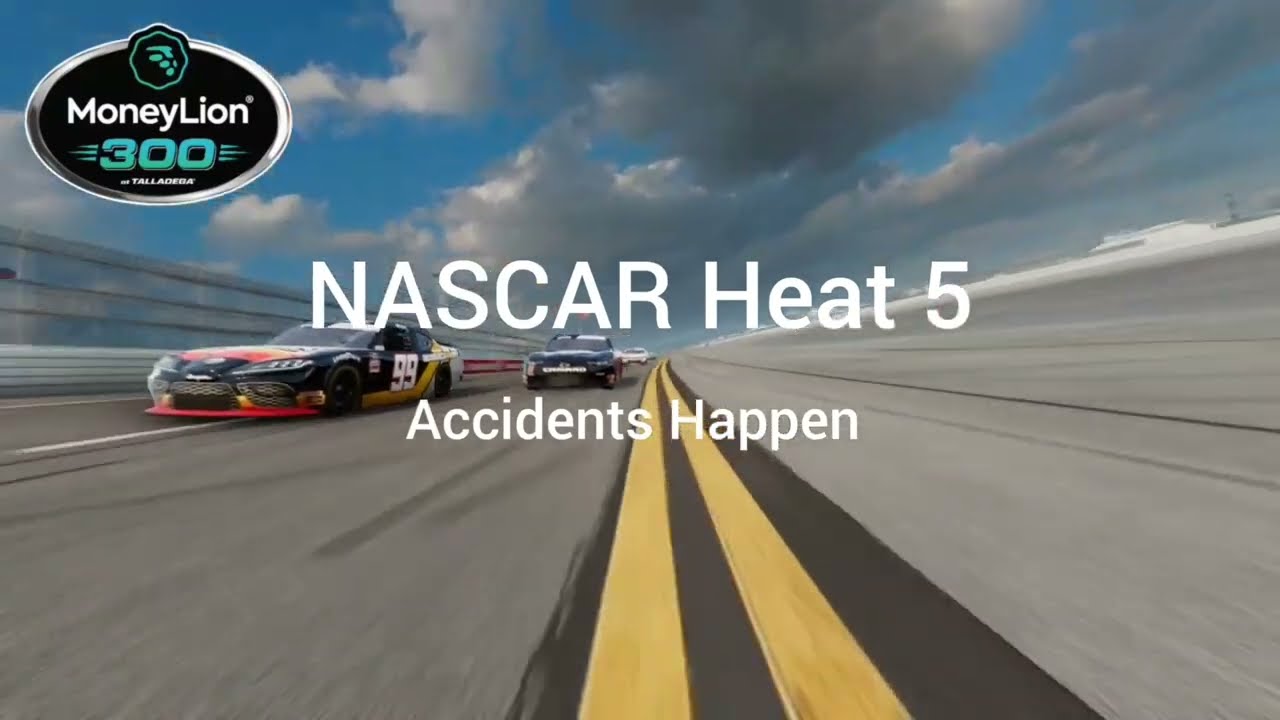The image is an outdoor photograph or poster of a NASCAR race taken from the center lane of the racetrack. At the forefront, the text "NASCAR Heat 5" is prominently displayed in white, narrow sans serif font, with the subtitle "accidents happen" just below it in a smaller but similar font. The viewer is positioned looking down a black pavement racetrack marked by two yellow stripes. On either side is a wider gray raceway surface.

The left side of the image features three NASCAR racing cars. The foremost car has the number 99 on its door and is adorned with blue and yellow stripes. Trailing behind it to the right is a blue car, and further back, a white car can be seen in the distance. A guardrail and a silver wall are also visible on the left-hand side of the image.

In the top left corner, an oval logo reads "Money Lion" in white letters on a black background, outlined with a silverish white border. At the top of this oval is a smaller black circle detail with a light blue lion logo. Beneath the text "Money Lion," the number "300" is displayed in turquoise blue with dashes on either side, accompanied by smaller unreadable white text below it.

The background of the image features a partly cloudy sky with patches of turquoise blue and some grayish rain clouds, setting the scene for this dynamic racing moment.